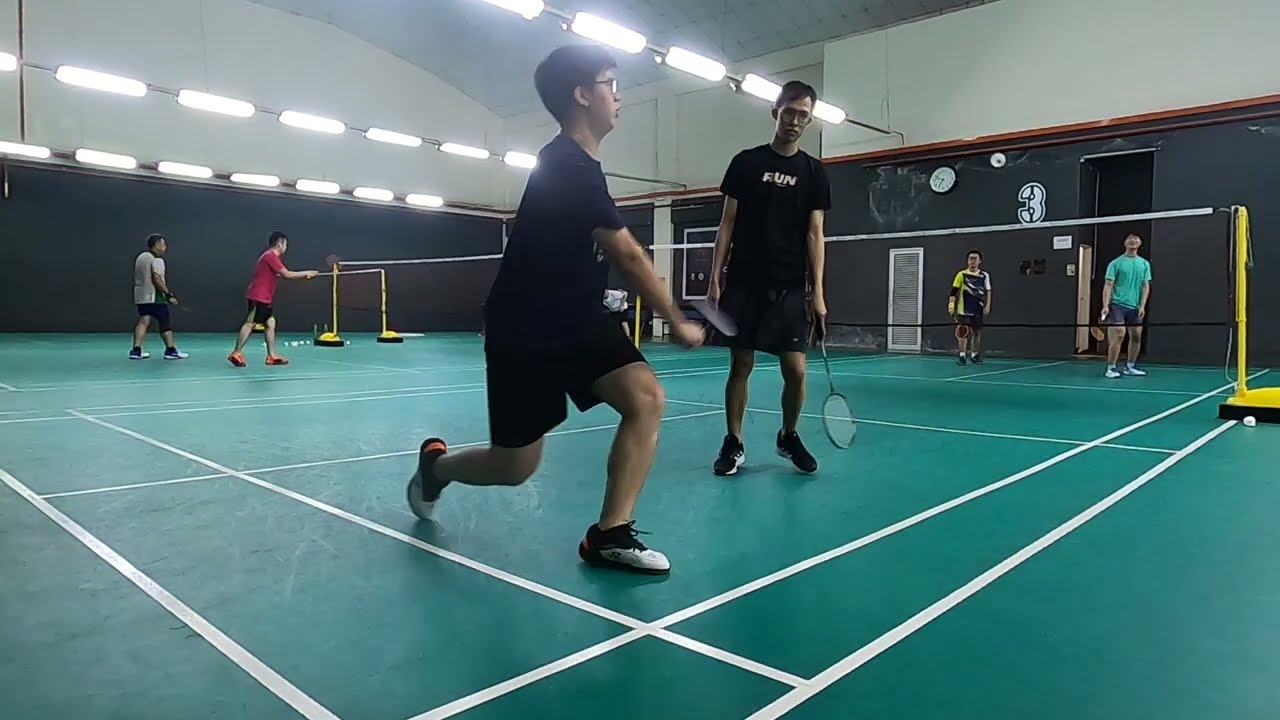An indoor badminton court houses two mirrored play areas marked by green flooring with white lines denoting boundaries. Two yellow pillars on each court hold a black and white net. The far wall features a dark gray lower half and a light gray or white upper half, with a visible clock. The gray ceiling has bright lights ensuring the space is well-lit. Closest to the camera are two men; one crouches slightly in black shorts, a black graphic t-shirt (possibly saying "fun" or "run"), black framed glasses, and black and white shoes. His partner, also dressed in black shorts, a black shirt, and black and white shoes, wears glasses and reaches for the shuttlecock. Their opponents wear yellow and mint green shirts. Other visible players include individuals in a red shirt and a white shirt on the left court, and a man in a light green shirt with his partner in a yellow shirt and dark vest on the right. A dark doorway is noticeable on the right, suggesting an exit.